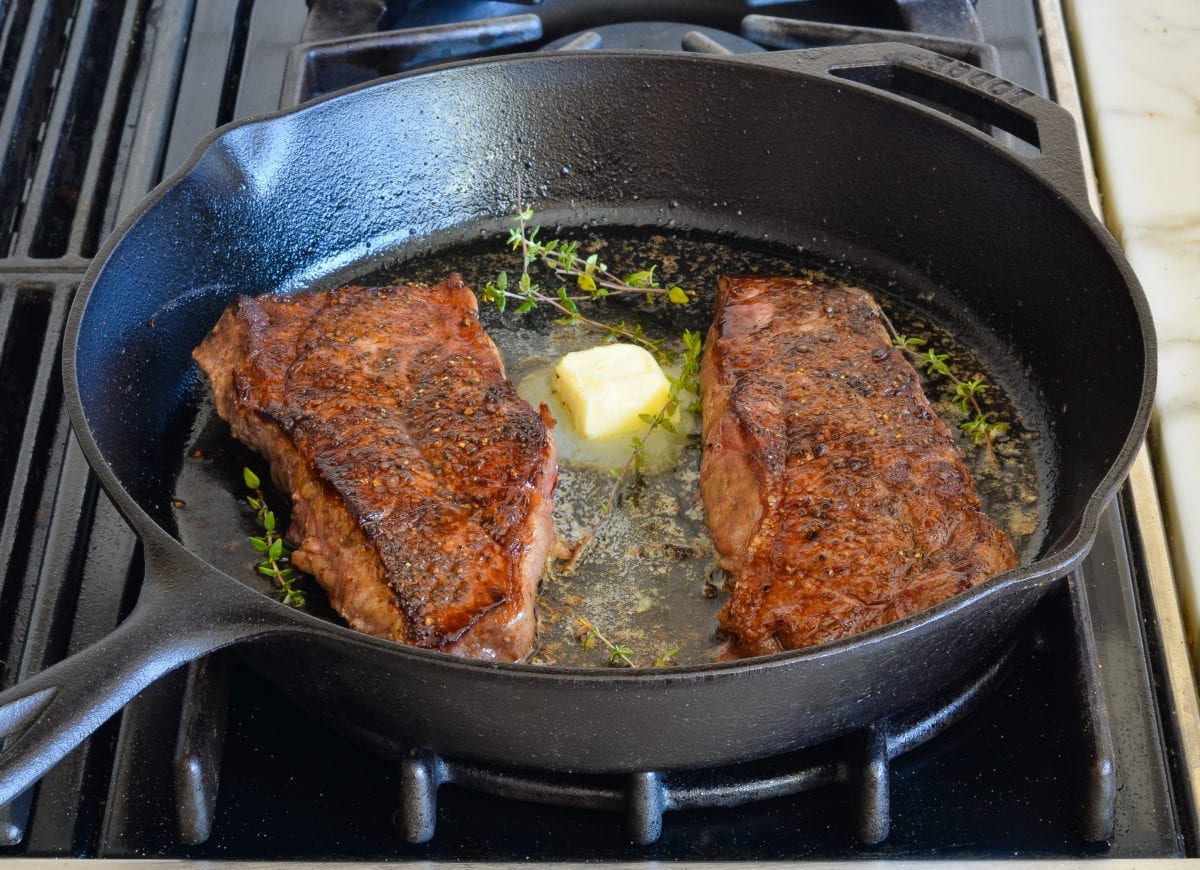The image depicts a pristinely maintained black cast iron skillet placed on a gas stovetop in a landscape orientation. The stovetop itself is glossy and well-kept, with another burner partially visible in the background. The skillet handle, which is slightly cut off, points diagonally to the left. It also features two lips for draining liquid. To the right, a thin strip of light off-white granite countertop, accented by a thin gold band separating it from the stovetop, is visible.

Inside the skillet, there are two well-browned, slightly charred fish steaks, seasoned generously and adorned with what appear to be thyme herbs. These herbs are sprinkled around and between the steaks. A melting knob of rich yellow butter sits in the middle of the pan, creating a mouth-watering blend with the herbs in the liquid surrounding the steaks. The overall effect of the image—with its rich browns from the steaks, green herbs, and the golden hue of the melted butter—evokes a strong culinary appeal, making it an enticing visual feast.